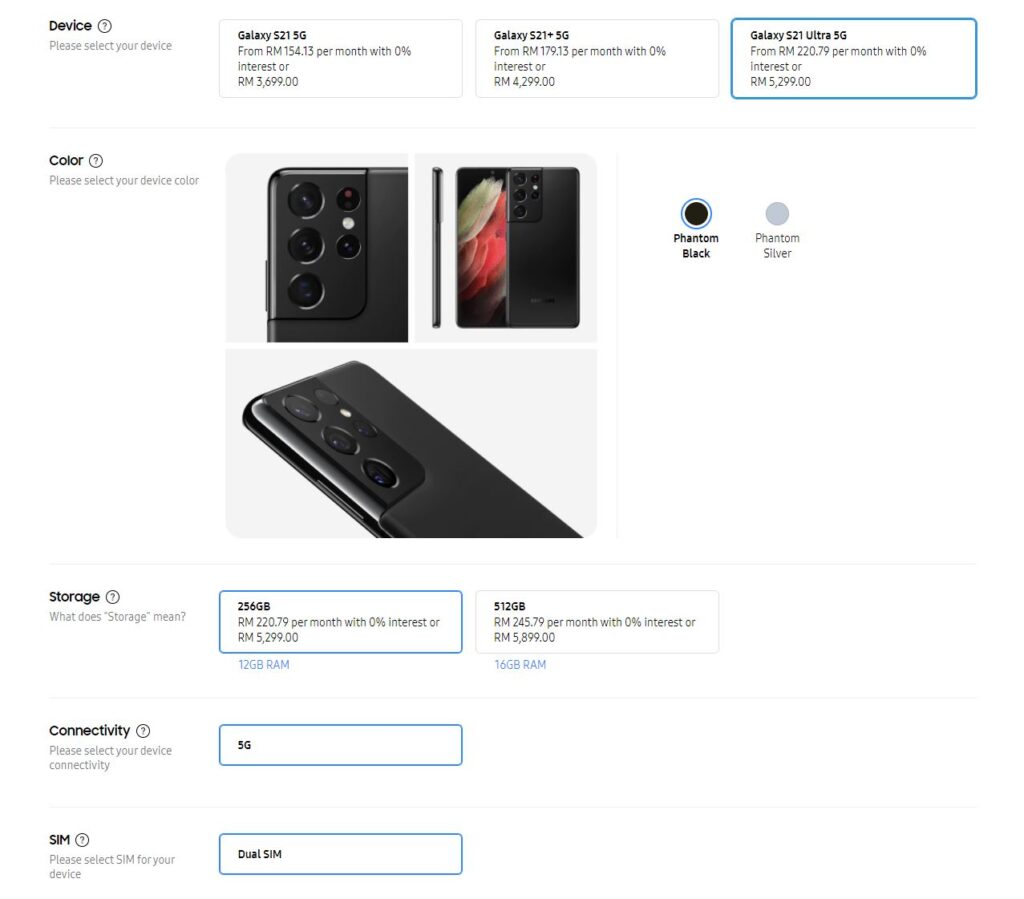A screenshot of a computer screen displays the selection interface for a Samsung Galaxy S21 5G series smartphone. The interface prompts the user with "Device? Please select your device" at the top. Various models, including the Galaxy S21, Galaxy S21+ 5G, and Galaxy S21 Ultra 5G, are listed. The S21 Ultra 5G model is highlighted, indicated by a blue border around its name. 

Further down, the selection menu includes a "Color" section where the chosen color, Phantom Black, is outlined in blue, while the alternative, Phantom Silver, remains unselected. Below that, there's a "Storage" section with a brief explanation titled "What does storage mean?". Two storage options are available: 256GB and 512GB. The 256GB option is selected, encircled by a blue outline. Additionally, preferences for 5G connectivity and dual SIM capabilities are highlighted, showcasing the user’s selections.